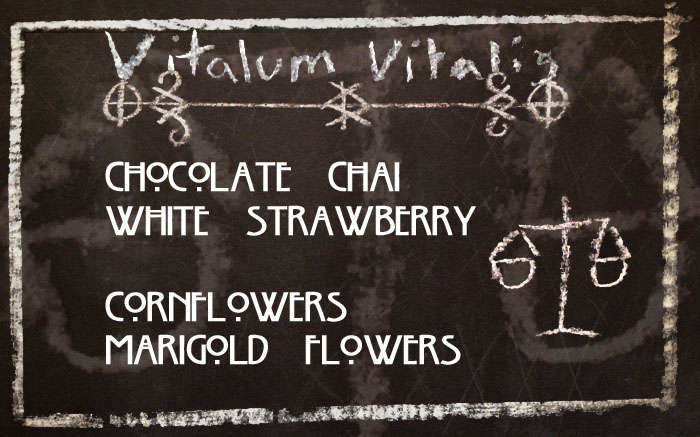The image features a black, chalkboard-style sign with a white chalk border that frames the entire design. At the top of the sign, the words "Vitalum Vitali" are prominently written in a hand-drawn, chalk-like font. Beneath this title, the sign lists several items: "Chocolate Chai," "White Strawberry," "Corn Flowers," and "Marigold Flowers." To the right of these lists, there is an illustration of a balanced scale with two baskets, indicative of equal weight, also drawn in white chalk. The overall aesthetic is very much in the style of a witchy or apothecary-themed chalkboard sign, with intricate details and careful linework.